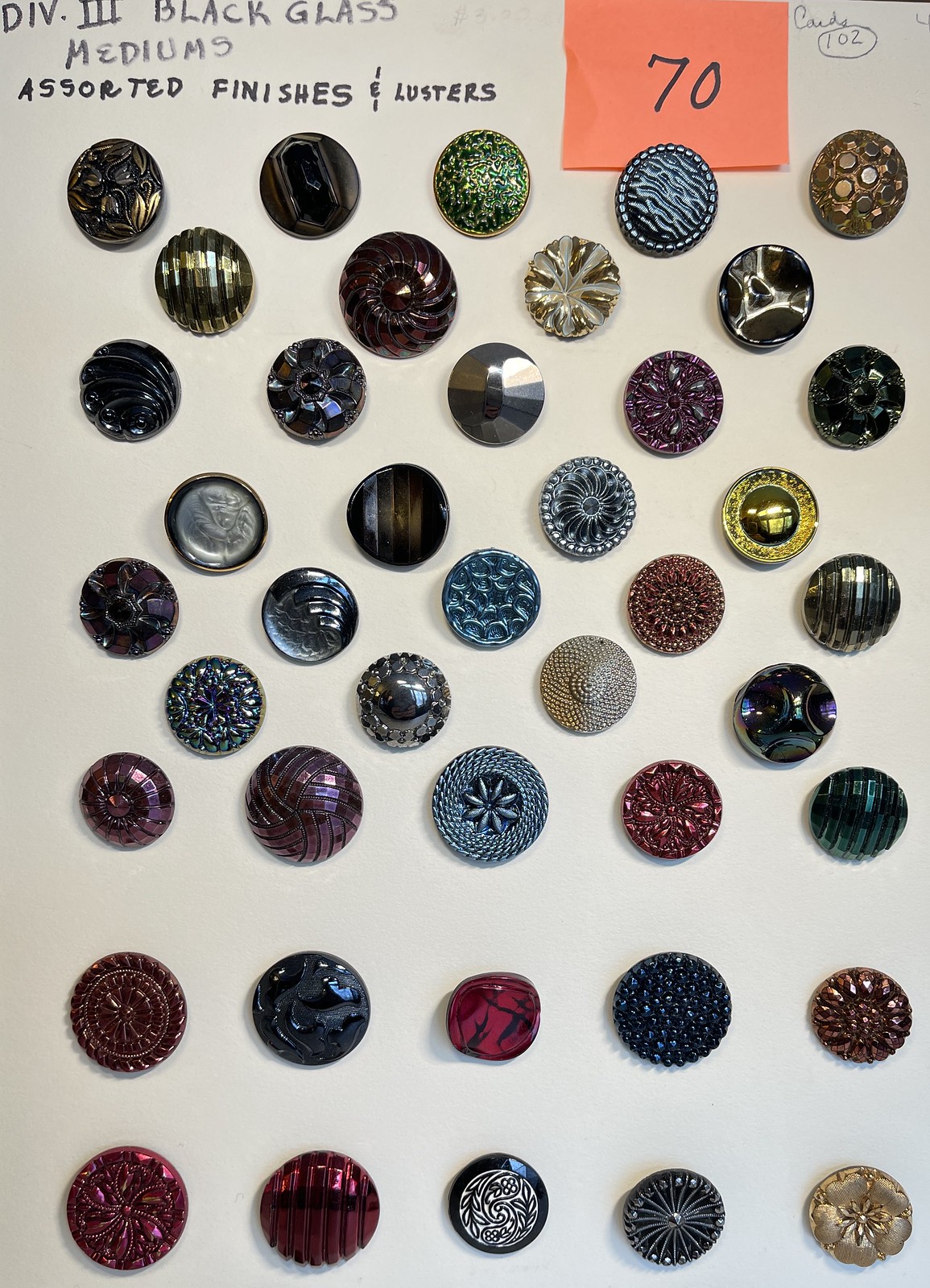The image depicts a vibrant assortment of glass buttons of various designs and finishes, displayed on a white background. At the top left corner, "Div 3 Black Glass Mediums Assorted Finishes and Lusters" is handwritten, with an orange sticky note beside it bearing the number 70 in black marker. This collection, likely intended to showcase 70 buttons, features an array of jewel-toned colors including reds, blues, yellows, and pinks. The buttons exhibit a mixture of shiny surfaces, reflecting light from the room. They are predominantly arranged in diagonal rows in the top two-thirds of the image, transitioning to two horizontal rows towards the bottom. The designs are diverse, ranging from simple round shapes to intricate floral and leaf patterns. Some buttons are metallic—gold, silver, and blue—while others appear to be stonelike, including a distinctive red and black one. The collection is visually striking, with each button offering unique textures and lusters.